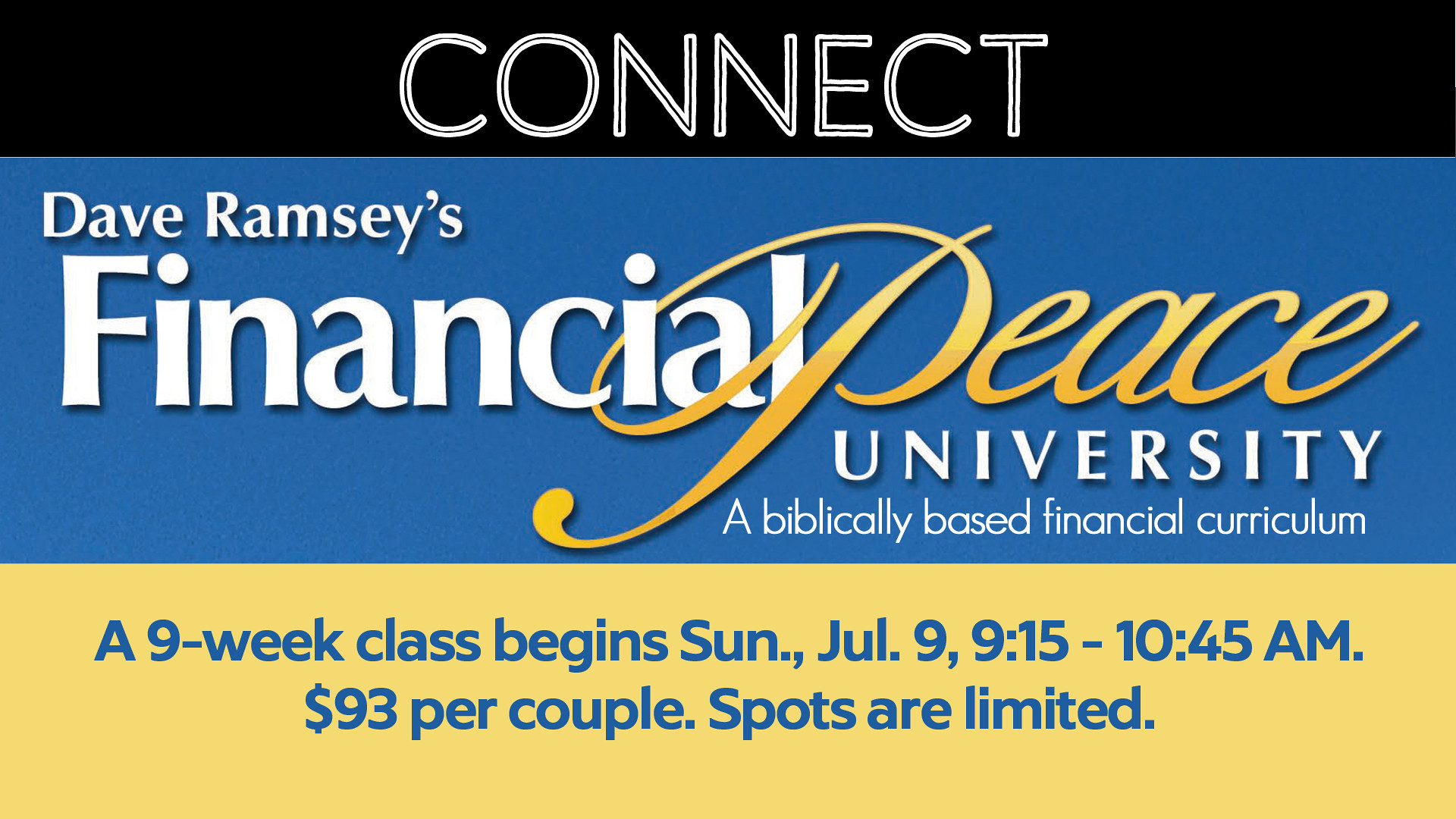This advertisement for a financial seminar features a structured design with distinct color blocks. At the top, there's a small black rectangular banner with the word "CONNECT" in bold, white, all-capital letters. Below this, a larger blue rectangular section prominently displays “Dave Ramsey’s Financial Peace University” with “Peace” highlighted in gold cursive font, followed by the phrase "a biblically-based financial curriculum" in white. The bottom section incorporates a smaller gold rectangular area with blue text providing further details: “A nine-week class begins Sunday, July 9, 9:15 to 10:45 a.m. $93 per couple. Spots are limited.”